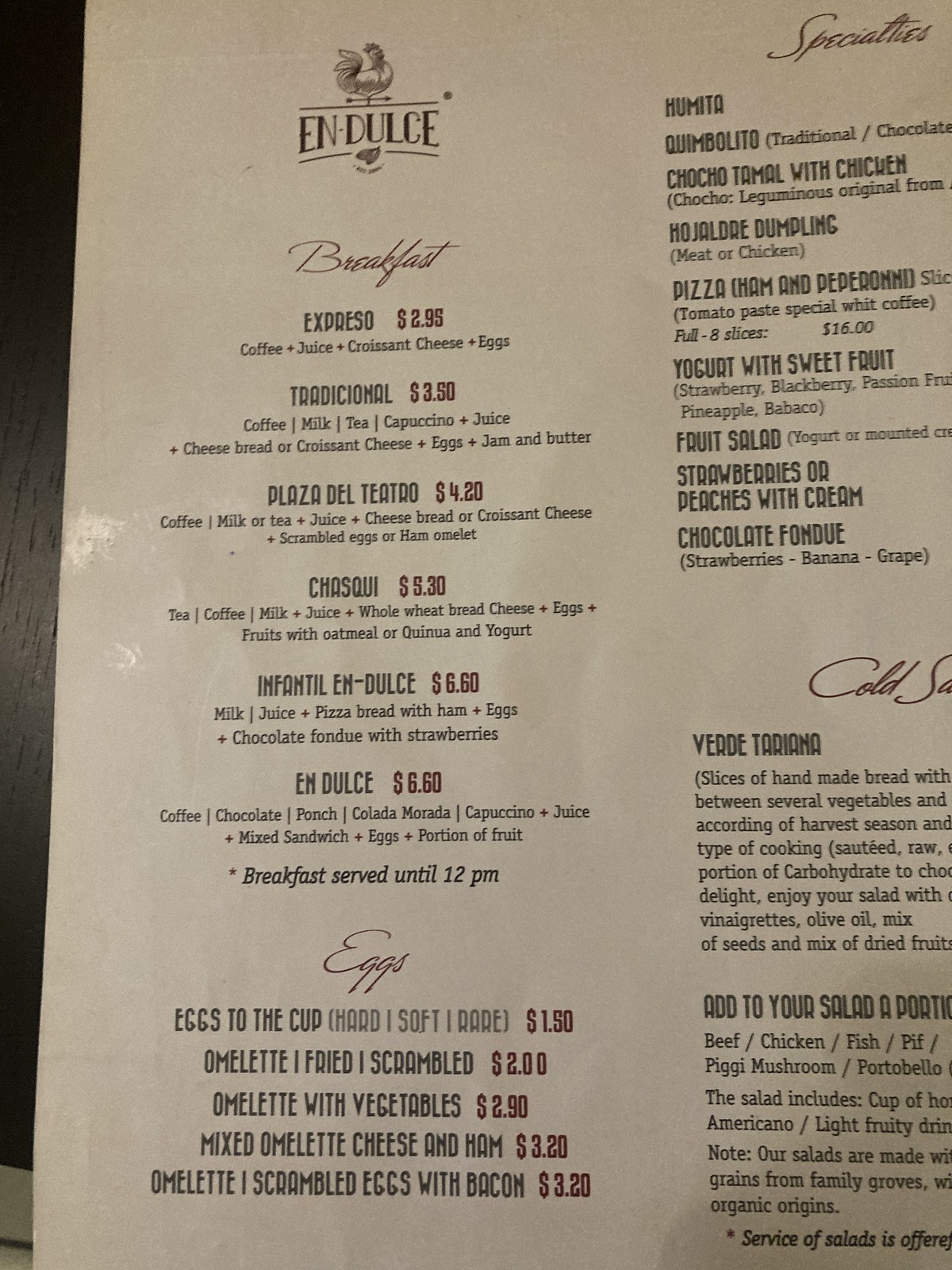Here's a cleaned-up and detailed descriptive caption:

---

This image shows a detailed menu from the restaurant Endulce. Centrally positioned at the top of the menu is the restaurant's name, "Endulce," accompanied by a small illustration of a chicken above it.

The menu offers the following breakfast options:

1. **Espresso ($2.95):** Includes coffee, juice, croissant, cheese, and eggs.
2. **Tradicional ($3.50):** Options include coffee, milk, tea, cappuccino, juice, along with cheese, bread or croissant, cheese, eggs, jam, and butter.
3. **Plaza del Teatro ($4.20):** Offers coffee, milk or tea, juice, cheese, bread or croissant, cheese, and a choice between scrambled eggs or a ham omelet.
4. **Chaski ($5.30):** Features tea, coffee, milk, juice, whole wheat bread, cheese, eggs, fruits with oatmeal, or quinoa and yogurt.
5. **Infantil Endulce ($6.60):** Comes with milk, juice, pizza bread with ham and eggs, and chocolate fondue with strawberries.
6. **Endulce ($6.60):** Includes coffee, chocolate punch, colada morada, cappuccino, juice, mixed sandwich, eggs, and a portion of fruit.

Breakfast is served until 12 p.m.

Under the breakfast section, there's a list of egg preparations:

1. **Eggs to the cup (hard, soft, rare) ($1.50)**
2. **Omelet, fried, scrambled ($2.00)**
3. **Omelet with vegetables ($2.90)**
4. **Mixed omelet with cheese and ham ($3.20)**
5. **Omelet or scrambled eggs with bacon ($3.20)**

In the top right corner, there's a section labeled "Specialties," featuring items such as:

1. **Humita**
2. **Quimbolito**
3. **Traditional chocolate**
4. **Choco tamal with chicken**
5. **Hojaldre (dumpling) with meat or chicken**
6. **Pizza with ham and pepperoni, tomato paste**

It also mentions a special wet coffee served with eight slices ($16), yogurt with sweet fruit including strawberry, blackberry, passion fruit, and pineapple, and a fruit salad with options of yogurt or mounted cream. Also listed are strawberries or peaches with cream, and chocolate fondue with strawberries, banana, and grape.

The bottom part of the menu contains further information, but it is obscured and not fully visible in the image.